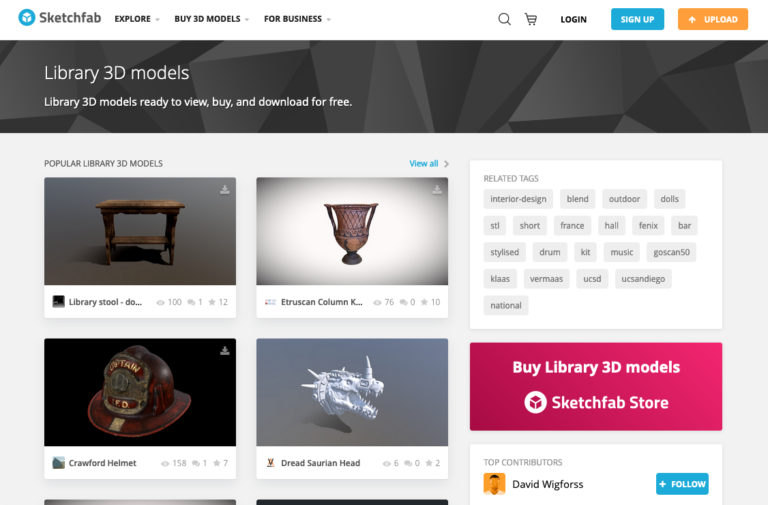Here's a detailed and cleaned-up caption for the described image:

---

In the upper left corner of the interface, the Sketchfab logo is displayed prominently. To the right of the logo, there are several interactive options including "Explore," "Buy 3D Models," and "For Businesses," each accompanied by a pulldown menu. Progressing further to the right, from the center to the right edge, the toolbar includes a search icon, a shopping cart, "Log In," a blue "Sign Up" button with white text, and an orange "Upload" button with white text.

Directly below this toolbar, a gray strip with a textured modulation spans the width of the screen. This strip contains the text: “Library 3D models, library 3D models ready to view, buy and download for free on the left.”

Beneath the gray strip, on the left side of the screen, there are four images arranged in a 2x2 grid. These images showcase popular 3D models from the library. The top left model is labeled "Library Stool," while the top right model is called "Trust in Column." The bottom left image features a fireman's helmet titled "Crawford Helmet," and the bottom right image is a dragon skeleton named "Dread Sardinian Head."

On the right side of the lower section, there are related tags listed, including "Interior Design," "Blend," "Outdoor," "Dolls," "STL," "Short," "France," "Hall," "Phoenix," "Bar," "Stylized Drum," "Kit," "Music," "Bermas," "USC," "ST," and "National."

---

This caption provides a clear and thorough description of the user interface and its elements.